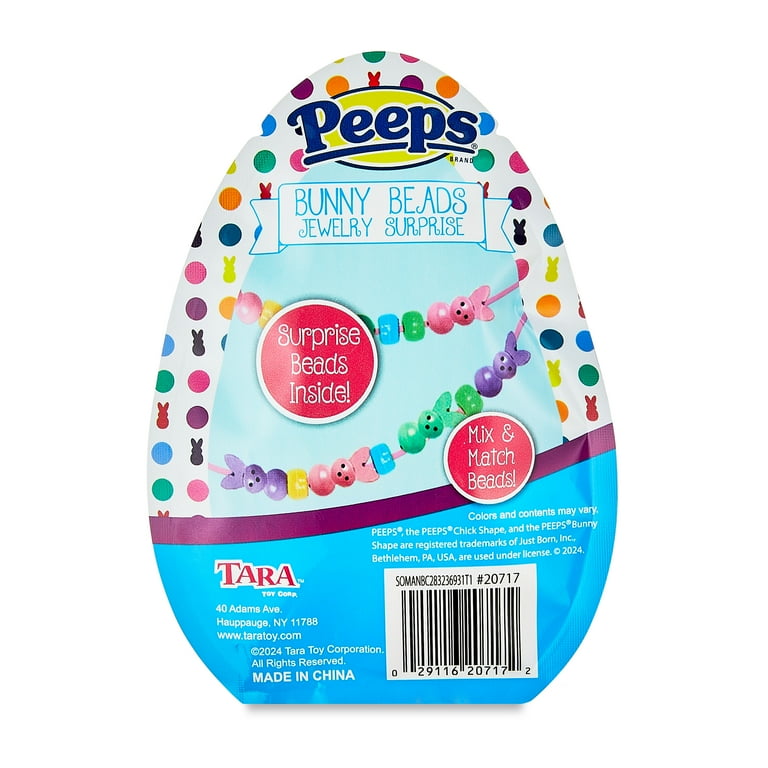This image features an egg-shaped packaging with a distinctive flat bottom, allowing it to stand upright. At the very top of the package is the recognizable Peeps logo in yellow and dark blue. Just below the logo, a white ribbon-like banner with blue text reads "Bunny Beads Jewelry Surprise." The upper section of the egg has a white background adorned with colorful circles and shapes of Peeps bunnies. 

Central to the design is a vibrant blue background with two strings of bunny-shaped beads displayed prominently. Towards the middle, two circular icons stand out: one pink circle with a white border containing the text "Surprise Beads Inside," and another pink circle that says "Mix and Match Beads."

The bottom half of the egg is predominantly blue and houses critical information. There is a barcode for scanning, followed by text stating "T-A-R-A, Made in China," and the address "Terra Corporation, 40 Adams Avenue, Hauppauge, New York, 11788." Additionally, it mentions that "Colors and contents may vary,” and highlights that the Peeps chick and bunny shapes are registered trademarks of Just Born Incorporated, Bethlehem, Pennsylvania, USA.